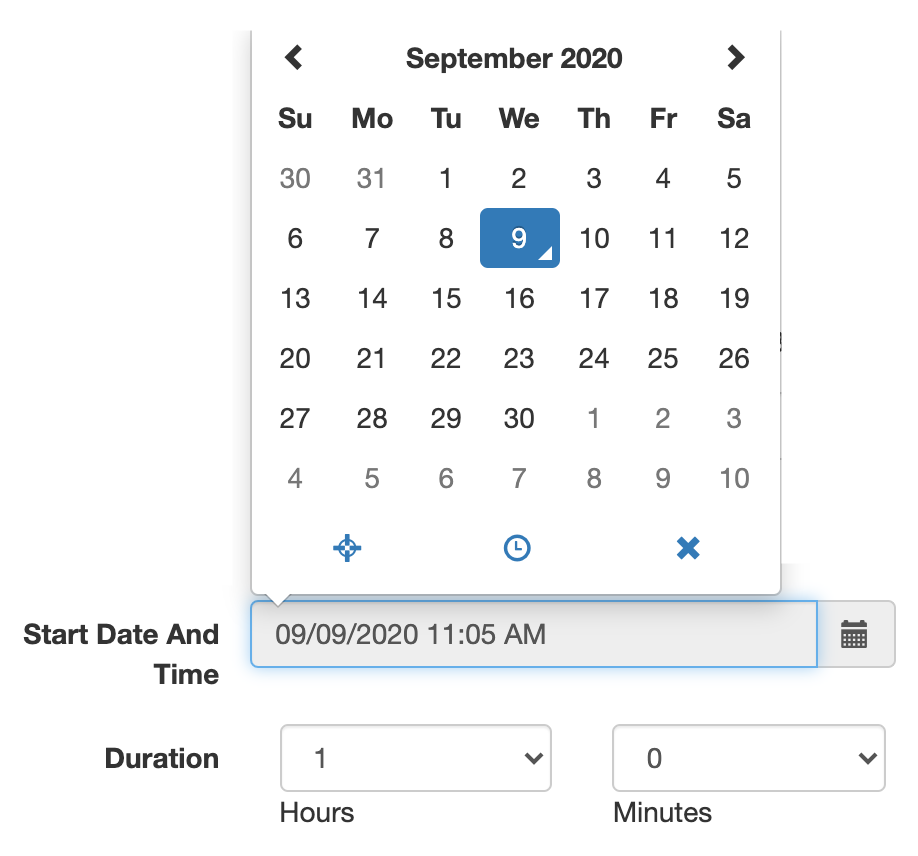The image shows a detailed calendar for September 2020. Each day of the week is meticulously listed: Sunday, Monday, Tuesday, Wednesday, Thursday, Friday, and Saturday. The days of the month are sequentially numbered from one to thirty, with specific circles highlighting certain dates, such as the eighth, tenth, and eleventh. An important notation indicates an event starting on September 9, 2020, at 11:05 a.m. The calendar is bordered in blue and features various kinds of days, possibly indicating different types of events or reminders. A toggle displays an hour, with an option to reset the minutes to zero. The intricate layout suggests a focus on scheduling and time management, emphasizing a one-hour concentration period adjusted with a dropdown to zero minutes.